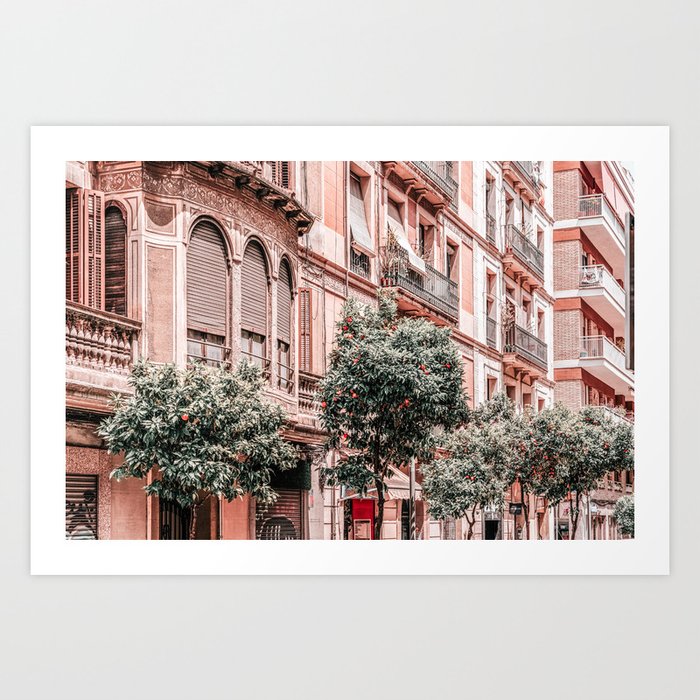This image captures a photograph of a red-brick high-rise building, possibly sourced from a postcard. The postcard itself is framed by a white border. The street is lined with similar high-rises, likely serving as apartments or living quarters, potentially featuring shops on the ground floor. In front of the buildings, trees add a natural element to the urban scene. The architecture evokes a French aesthetic with arched windows, ornate balconies, and a mixture of white and red brickwork. Various blinds hang outside the windows, contributing to the vibrant residential ambiance.